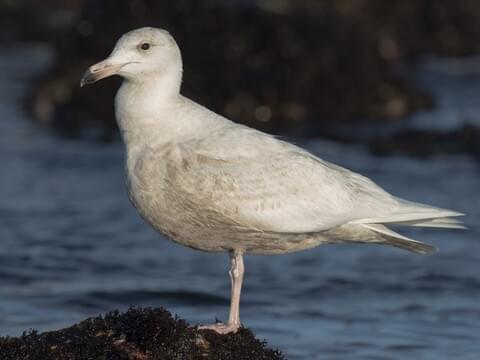A weathered seagull, its dirty white feathers streaked with shades of tan and gray, stands solitary on a rock covered in black moss. The bird's figure is prominently displayed against a blurred background of choppy dark water and indistinct rocky formations. The water is dark, rippling under apparent wind, signifying a rough day at sea. The seagull, facing to the left, exhibits signs of neglect; its stomach is stained, and its pallid legs contribute to its overall sickly appearance. The bird's tired eyes and a distinctive black-tipped beak add to its disheveled look. Only one leg is visible, as the other is positioned behind, emphasizing the bird's side profile. The image's quality is somewhat blurred, adding a sense of melancholic isolation to the scene.